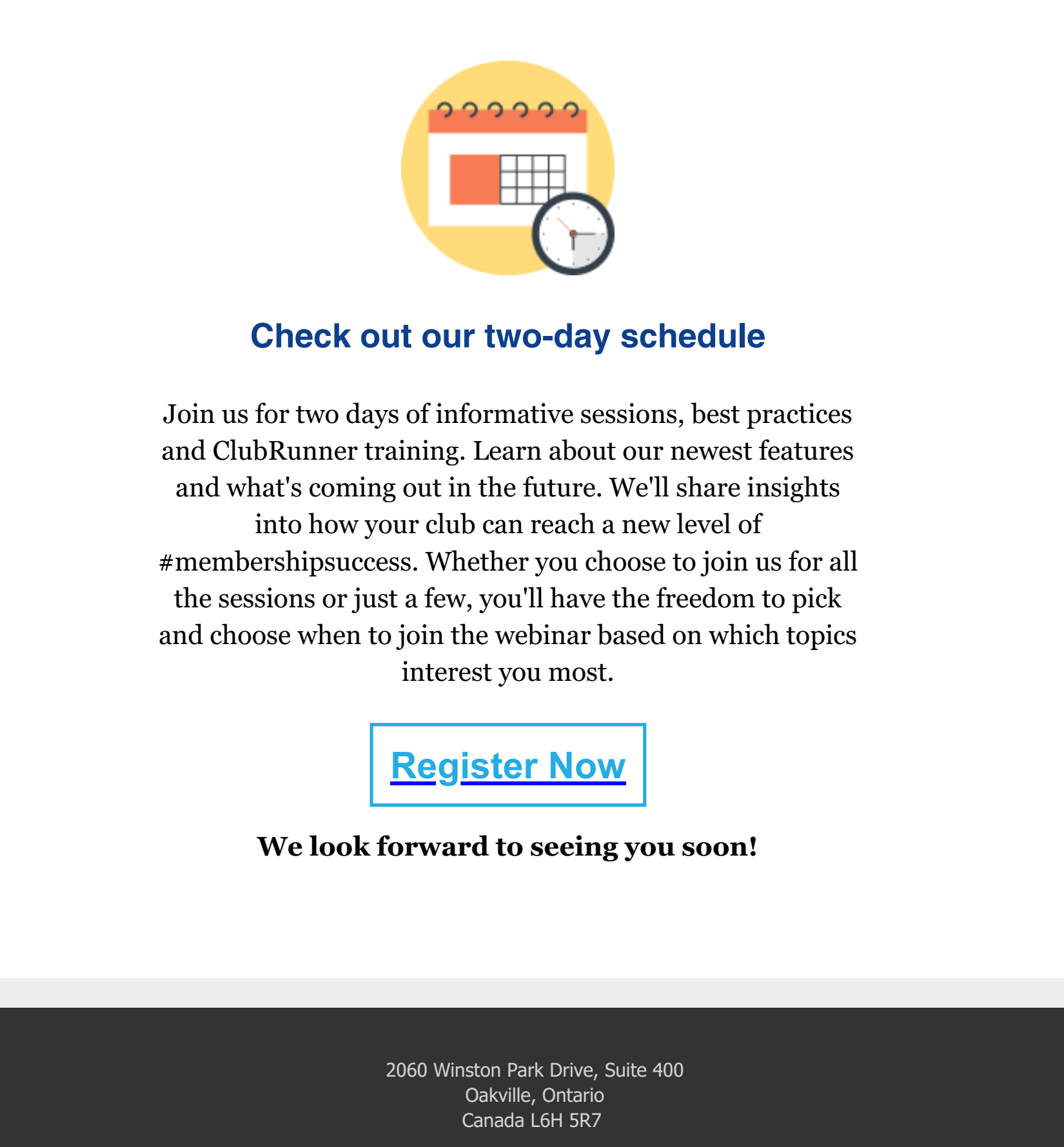The image features a vertically-oriented rectangle with a white background. At the top center of the image is a yellow circle containing a calendar icon in orange, white, and black. In the bottom right corner, there is a clock with a black frame and a white face, displaying the time 6:15.

The text begins with a blue section that reads, "Check out our two-day schedule." Below it, in black font, it says, "Join us for two days of informative sessions, best price practices, and ClubRunner training. Learn about our newest features and what's coming out in the future. We'll share insights into how your club can reach a new level of #membershipsuccesses. Whether you choose to join us for all the sessions or just a few, you'll have the freedom to pick and choose which webinars to attend based on your interests."

Following this, there is a white button with a turquoise outline that says "Register Now" in turquoise text. A blue line is situated beneath the button, and below the line, a black bolded message reads, "We look forward to seeing you soon."

At the bottom of the image, there is a thin gray strip followed by a thick black strip. In the thick black strip, an address in white font states, "2060 Winston Park Drive, Suite 400, Oakville, Ontario, Canada, L6H 5R7."

This detailed caption summarizes the event's advertisement and provides information regarding the event's purpose, schedule flexibility, and registration details.